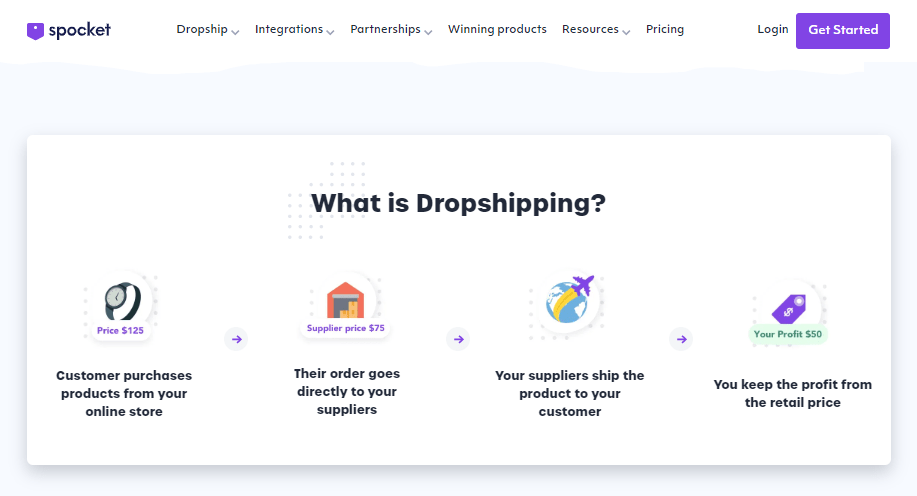The image appears to be a screenshot of a dropshipping platform interface on a computer screen. In the upper left corner, there is a purple shield icon next to the word "Sprocket." Moving across the top of the screen, there are navigation tabs labeled "Dropship," "Integrations," "Partnerships," "Winning Products," "Resources," and "Pricing." On the far right side, there are options for "Login" and a purple "Get Started" button.

The background is gray, with a large white rectangle prominently displayed in the center. Inside this rectangle, the text "What is Dropshipping?" is centered at the top. Below this header, four icons are lined up horizontally across the screen, each representing a step in the dropshipping process.

1. The first icon is a watch labeled "Price $125," with the text "Customer purchases products from your online store" beneath it. An arrow points to the right.
2. The next icon is a picture of a house labeled "Supplier price, $75," with the description "Their order goes directly to your suppliers." Another arrow points to the right.
3. The third icon is an image of a globe with a purple airplane flying across it, accompanied by the text "Your suppliers ship the product to your customer." An arrow points to the right.
4. The final icon is a circle with a purple price tag, labeled "Your profit, $50." The description below this icon reads "You keep the profit from the retail price."

Overall, the screenshot clearly outlines the dropshipping process step-by-step with visual aids and accompanying text.